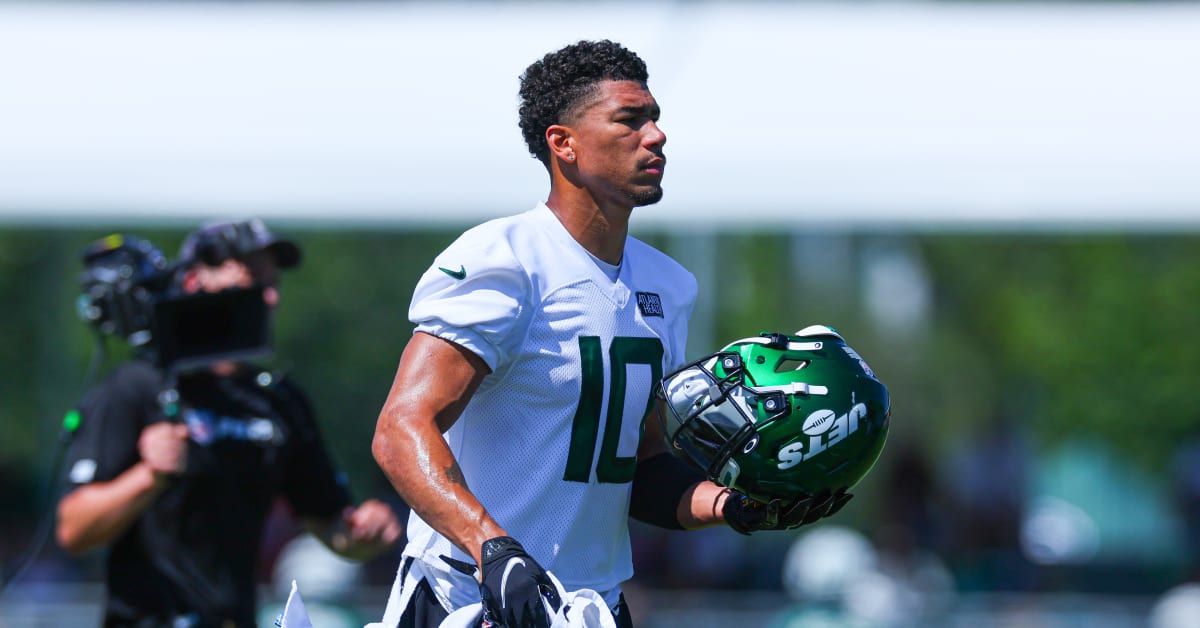In this horizontally oriented photograph, we see a young African-American football player, possibly in his 20s or 30s, identified as Alan Lazard, the wide receiver for the New York Jets. He is captured from the waist up, centered in the frame, gazing off to the right. He is dressed in a white Jets jersey with the number 10 and a green Nike logo, indicating it’s a practice session rather than a full-contact activity. In his left hand, he holds a green helmet with a white Oakley "O" logo and the word "Jets" emblazoned across it. He also sports black Nike gloves. Lazard appears fit and muscular, with visible sweat suggesting physical exertion.

To the left of the frame is a slightly blurry cameraman with white skin, holding a video camera on his shoulder, likely documenting the practice. The background is out of focus, with hues of green and white, suggesting a stadium or practice field setting. The overall scene captures the intensity and dedication of the player during what appears to be a moment of respite.